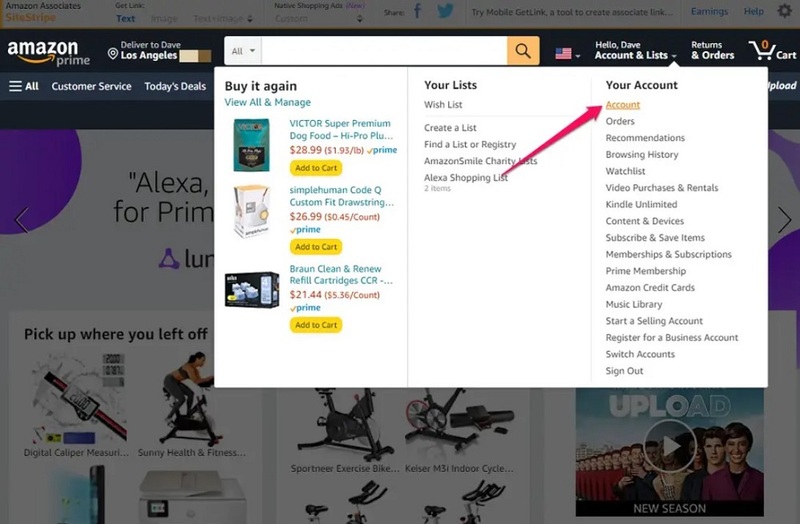The screenshot shows the Amazon website homepage, prominently displaying a white pop-up menu that has been pulled down from the "Hello, Dave" section located under "Accounts & Lists" on the top right corner. The main background of the page is grayed out to highlight the active menu. 

On the left side of the screen, the website header includes text indicating: "Amazon Prime, deliver to Dave, Los Angeles." Below, there is a "Buy It Again" section with options such as "View All and Manage." Displayed products include items like "Victor Super Premium Dog Food, High Pro Plus" priced at $28.99, with an "Add to Cart" button, and "Simple Human Code Q Custom Fit Drawstring" included as well.

In the center of the pop-up menu, several sections are visible: "Your Lists" features options to create or find a list or registry, access the Amazon Smile Charity List, and check the Alexa Shopping List. A red arrow at the bottom of the "Alexa Shopping List" points towards the "Your Account" section. This section contains a variety of links in orange text, including "Orders," "Recommendations," "Browsing History," "Watch Video Purchase and Rentals," "Kindle Unlimited Content and Devices," "Schedule," "Subscribe & Save Items," "Membership and Subscriptions," "Prime Membership," "Amazon Credit Cards," "Music Library," "Start a Selling Account," "Register for a Business Account," "Switch Accounts," and "Sign Out." The prominent red arrow encourages navigation to "Go to Account."

Overall, the detailed navigation options and purchasing suggestions encapsulate the comprehensive user interface designed to streamline user interactions on Amazon.